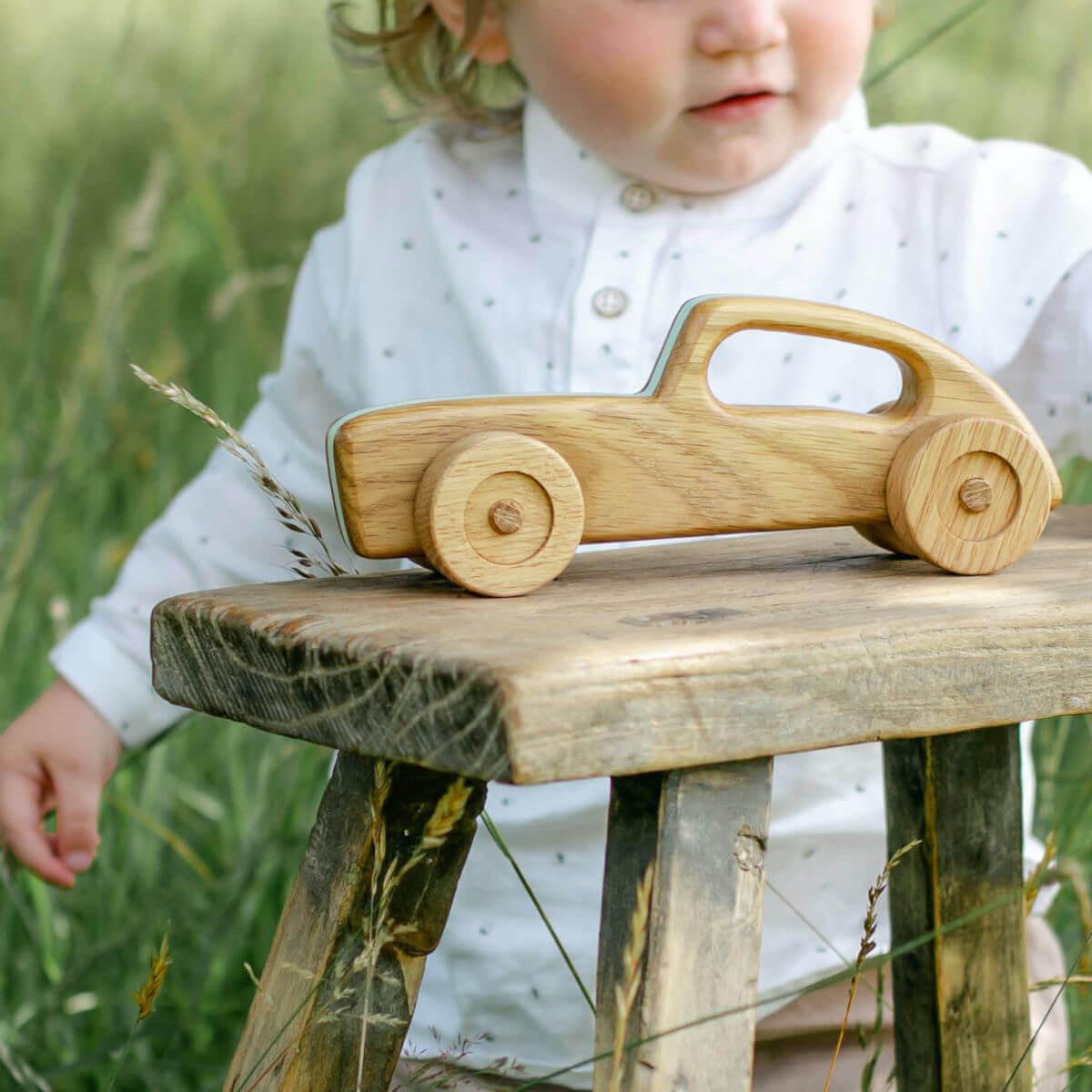In this detailed and vibrant photograph, the focal point is a meticulously hand-carved wooden car, proudly displayed on a brown woodworking bench situated in a grassy field. The car, crafted from a single piece of wood, features smoothly rounded wheels attached with central hubs and a handle-style cutout where the window would be, showcasing excellent craftsmanship. The image captures a glimpse of a young toddler girl standing slightly behind the car, with her chubby cheeks and lips in focus, wearing a white blouse adorned with little black dots. Her attire and rosy cheeks add a delicate touch of color to the scene dominated by natural tans, browns, and greens. The photograph, framed in a square format, emphasizes realism and detail, centering on the wooden toy car, which is oriented with its front facing left. The girl's position, mid-nose to hip length visible, offers a soft, blurred background, bringing the woodwork's detail into sharper relief. The entire scene evokes a sense of rustic simplicity and innocent childhood, making the wooden car the undeniable star of the composition.